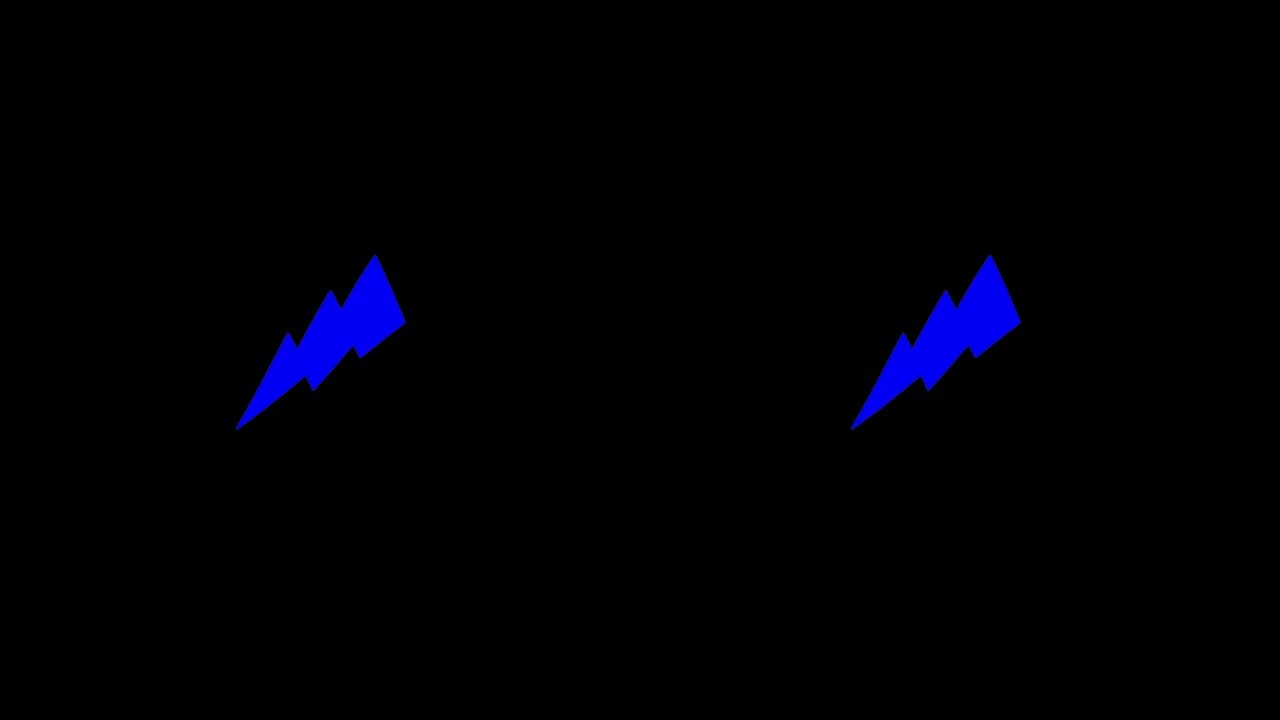The image is a rectangular photograph with a completely black background featuring two vivid royal blue lightning bolts. Each lightning bolt, about an inch long, is tilted downward to the left, with their thicker sectors oriented towards the top right corner. Positioned horizontally across the central height of the frame, the bolts are spaced out in the image’s left and right thirds, leaving a significant gap of black space in the middle. The lightning bolt on the left is positioned slightly towards the right from the left border, while the one on the right is slightly towards the left from the right border, without touching either edge. The bolts appear identical, making them look manipulated or duplicated, and the simplicity of the black and blue contrast draws the viewer's attention solely to them, creating a stark and graphic visual effect.